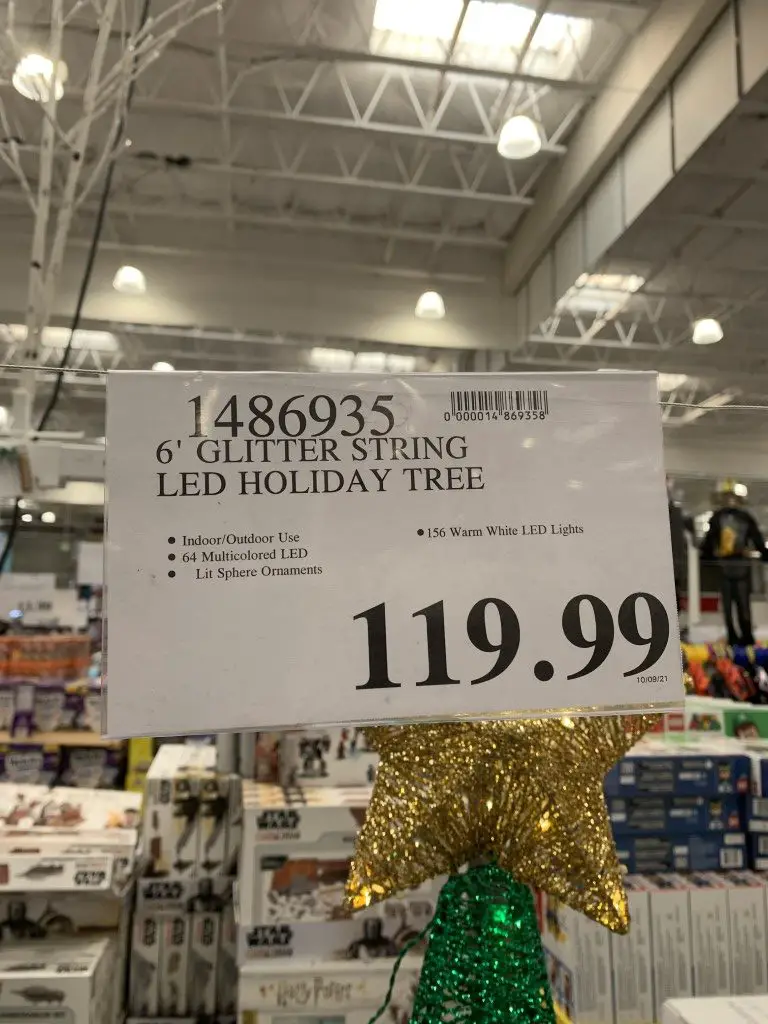The photograph captures the bustling interior of a warehouse-style bulk shopping store, reminiscent of Sam's Club or Costco, characterized by its high ceilings supported by white metal structures. In the background to the left, a white tree-shaped decoration is prominently displayed, enhancing the festive atmosphere. The scene is enlivened by a stack of popular Star Wars and Harry Potter toys arranged centrally. In the bottom section of the image, a striking green and yellow foil holiday tree, topped with a gold star, adds to the seasonal decor. Above this festive ornament, a detailed white sign reads: "1486935 6-foot Glitter String LED Holiday Tree. Indoor/Outdoor Use. 64 Multicolored LED Lit Sphere Ornaments and 156 Warm White LED Lights." This descriptive sign provides shoppers with specific product information, contributing to the organized and informative layout of the store.